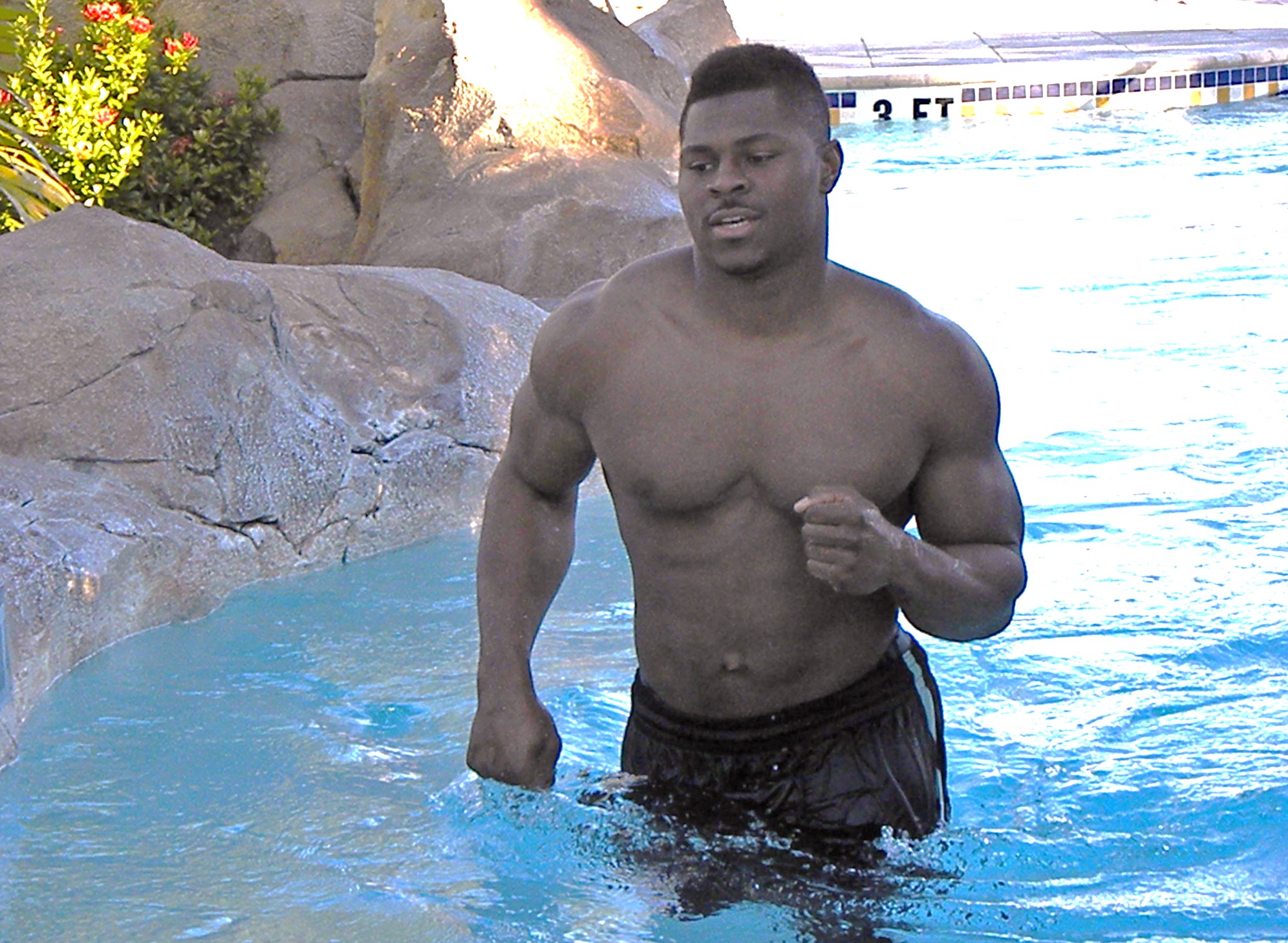In this vibrant photograph, a young, muscular man with short black hair and a very short moustache is captured standing in a bright blue swimming pool, wearing black swim shorts. The man, who appears to be of African descent, has dark skin and is topless, showcasing his well-defined six-pack and muscular arms. One of his arms is bent with a fist up to his chest, while the other is positioned behind him, giving the impression that he is either running or dancing in the water. To the top left of the image, there are rocks adorned with green shrubs that have striking red flowers. The pool edge, visible at the top of the image, features a blue-tiled border interspersed with small blue, orange, and white squares. Prominently displayed on the ledge above the pool, a white sign with black text indicates the water's depth as "3 feet." The scene is bathed in sunlight, enhancing the vivid colors and lively atmosphere.